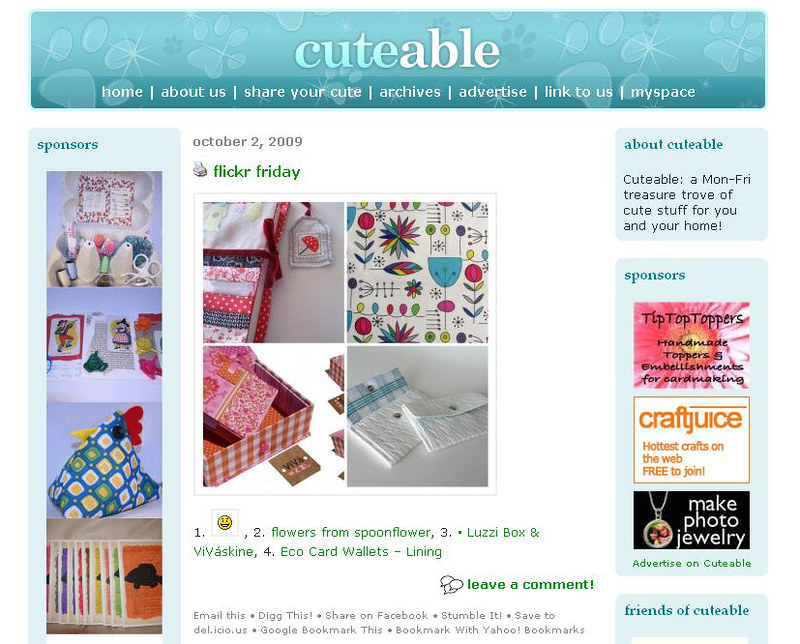The image is a detailed screenshot of a website named "Cutable," featuring a blue banner at the top with superimposed paw prints. Beneath the banner, there is a navigation menu with options: Home, About Us, Share Your Cute, Archives, Advertise, Link to Us, and MySpace. The central content includes a blog post dated October 2nd, 2009, titled "Flickr Friday," showcasing a two-by-two grid of close-up photos featuring various fabric projects. These photos include items such as a fabric book cover, handmade napkins, and white purses. Each photo is captioned and numbered: 1 with a smiley face image, 2 labeled "Flowers from Spoonflower," 3 titled "Loozy Box from Viviskin," and 4 named "EcoCard Wallets - Lightning." The site has sponsor sidebars on both the left and right, filled with advertisements and images of handmade crafts. On the right sidebar, there is a section titled "About Cutable," describing it as a Monday through Friday treasure trove of cute items for home and personal use. Below the grid of images, there is a "Leave a Comment" section, encouraging user interaction. The bottom of the page also has options for email, sharing on Facebook, and other additional information.